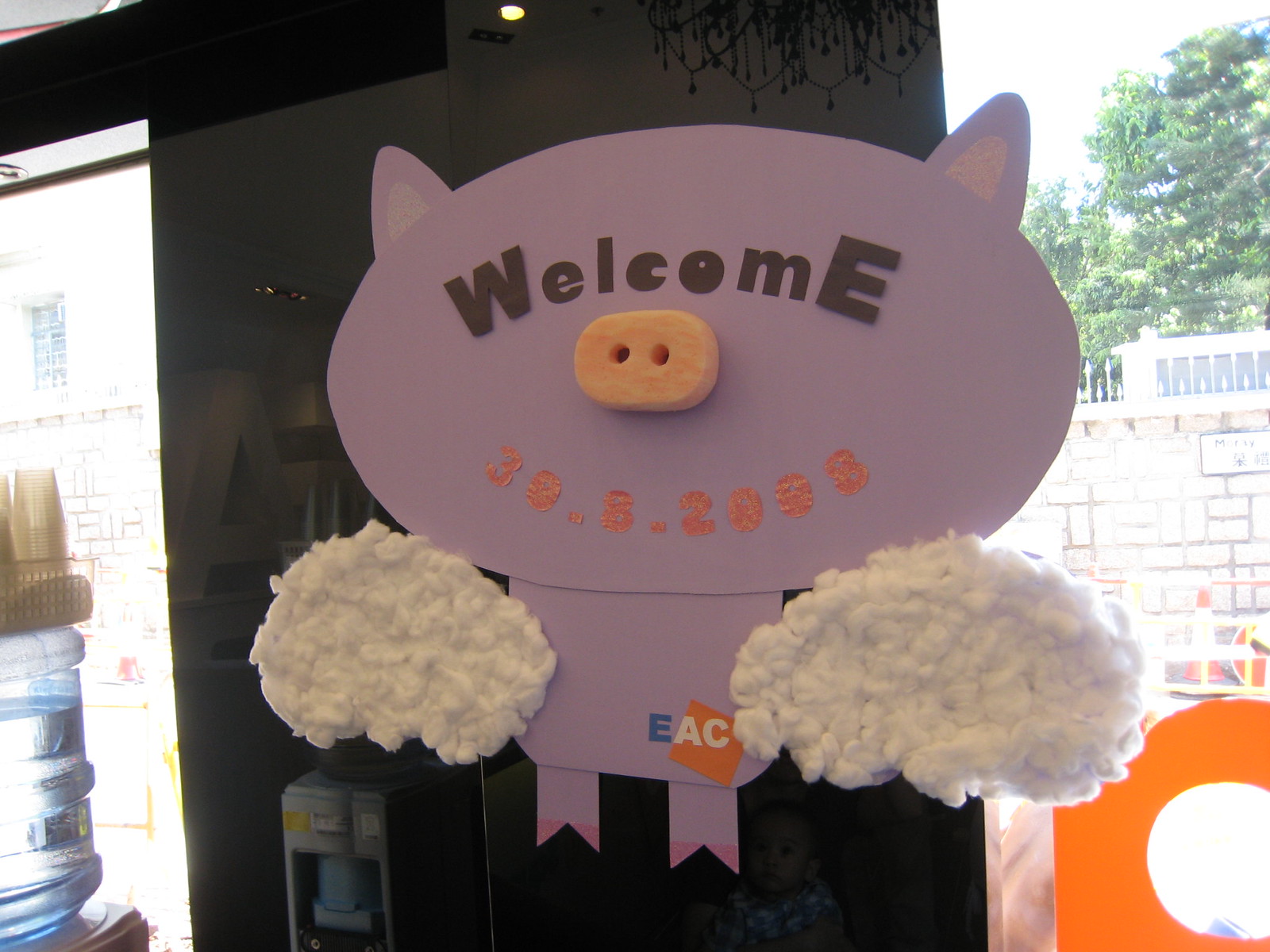The image depicts an indoor scene looking out through windows to an outdoor area with a brick wall and trees in daylight. The focal point is a purple paper cutout shaped like a pig mounted on the brick wall outside. The pig graphic, simple and child-like, has a large circular head with a button-like nose featuring two holes, and "WELCOME" written where its eyes would be. Below, numbers such as 388, 3862098, or 2008 and the letters EAC are displayed, the latter inside an orange square. The pig’s hands or front legs hold soft, pom-pom-like objects. Accompanying the pig are illustrations of clouds to its left and right. The setting suggests a playful, educational environment, possibly a school, daycare, or library. Inside the room, there's a water cooler on the left with a water bottle on top.